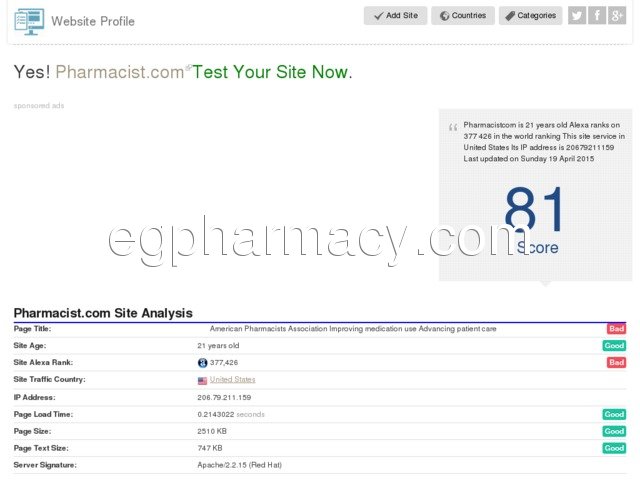Screenshot of a Website Performance Analysis for Pharmacist.com

This detailed screenshot provides an in-depth analysis of the website Pharmacist.com, as evaluated by a site testing service. The primary focus is on various performance metrics displayed in a well-organized layout with color-coded statuses for quick assessment.

At the top, the interface includes profiles for adding sites, countries, and categories, each marked with representative icons. A prominent call-to-action button in green urges users to "Test Your Site Now". 

There is also a section for sponsored ads, although specific advertisements are not visible in this screenshot.

The website's overall performance score is displayed in large blue numbers, showing '81'. Accompanying this is text detailing the site’s age of 21 years, an Alexa site rank of 3777,426, and the site's IP address: 206.79.211.159. 

Key data points include:
- Last updated: April 19, 2015.
- Organization: American Pharmacists Association, known for improving medication use and advancing patient care.

Performance metrics are highlighted with badges indicating their status:
- Site Age: 21 years – Status: Good (Green badge)
- Alexa Rank: 3777,426 – Status: Bad (Red badge)
- Site Traffic (Country: United States) – Status: Good (Green badge)
- IP Address: 206.79.211.159
- Page Size: 2510 kilobytes – Status: Bad (Red badge)
- Load Time: 0.2 seconds (or 0.214322 seconds) – Status: Good (Green badge)
- Server Type: Apache/2.2.15 (Red Hat) – Status: Good (Green badge)

The design of the analysis page aims to provide a quick and clear summary of the website's performance, with key metrics and their respective statuses prominently highlighted in different colors. The overall theme is functional yet informative, designed to offer an at-a-glance understanding of the site's health. 

It is worth noting that a large watermark reading "pharmacy.com" is centered on the image, suggesting an attempt to underscore a point about another pharmacy-related site, possibly for comparison purposes.